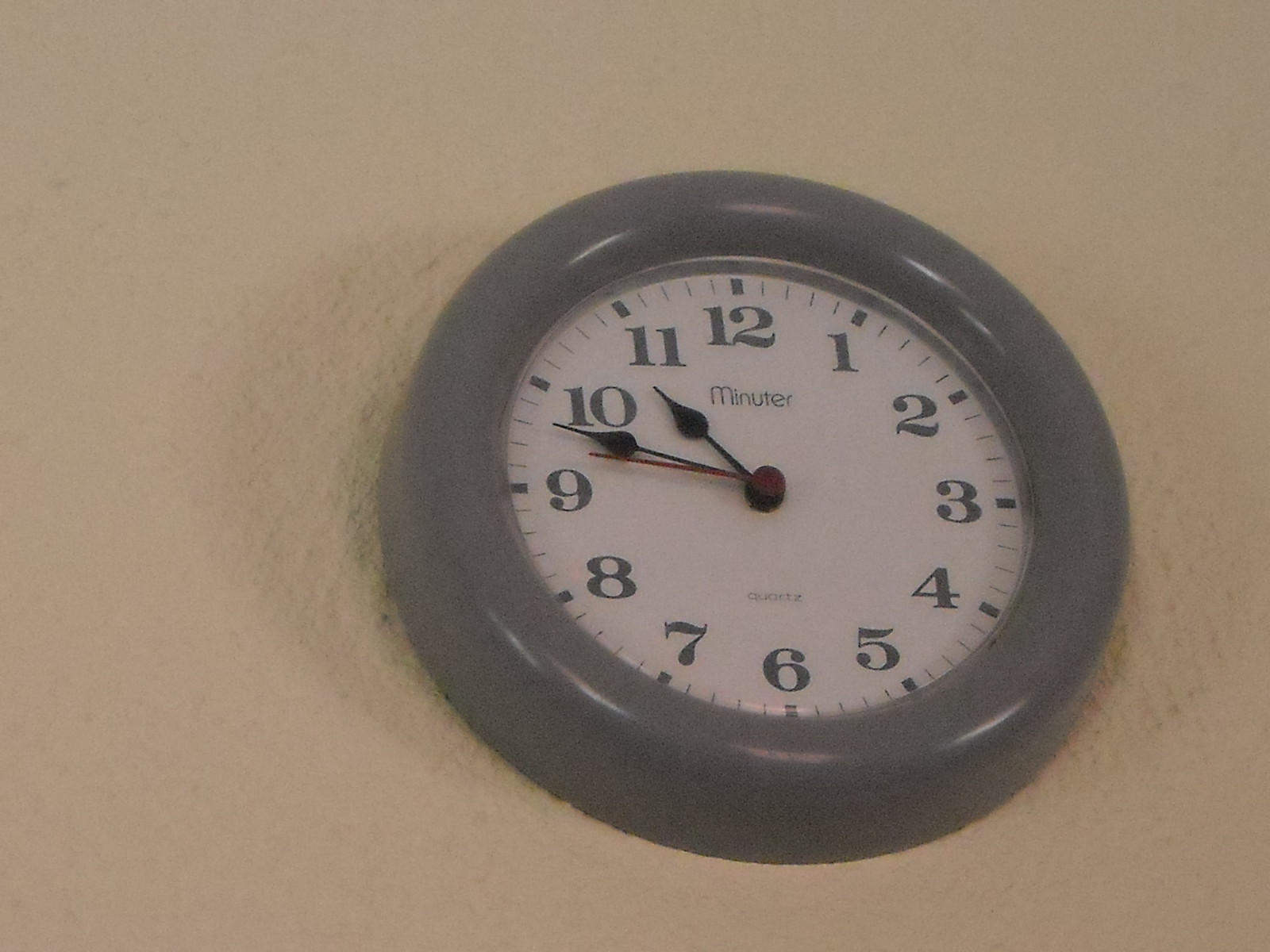In this detailed black-and-white photograph, a plain, white-painted ball sits against a background of old, chipped wallpaper, marked by the telltale smudges and tiny dings accumulated over years of contact. The ball shows signs of wear with visible scuffs and minor imperfections. Dominating the center but slightly offset to the right, an unmistakably vintage clock from the 1980s draws attention. The clock, encased in a basic, potentially black or red plastic frame, features bold numbers reminiscent of the Times New Roman font. The clock face is marked by three distinct hands: a big hand, a little hand, and a red second hand, which currently points to approximately 12 minutes to 11. The simplistic, quartz clock bears the inscription "Minutes," highlighting its utilitarian design.